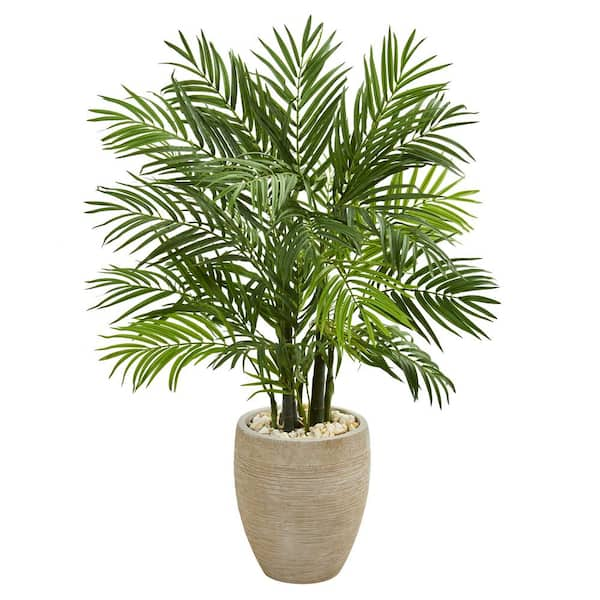This image depicts a tropical potted plant, likely intended for advertisement. The plant is housed in a large beige or tan ceramic, possibly terracotta, vase. The top of the planter is filled with white rocks, a common practice for drainage. The plant prominently features lush, variegated green foliage, with shades ranging from dark to light green. The leaves have a fern-like or palm frond appearance, with multiple fan-like structures and many elongated leaves extending from each branch. The plant comprises several thick stalks rising from the base, indicating a healthy and well-kept specimen. The photograph is taken against a plain white background, offering no additional context or scale, but it suggests that the planter itself is about one to two feet tall, with the plant extending a few feet beyond that height.